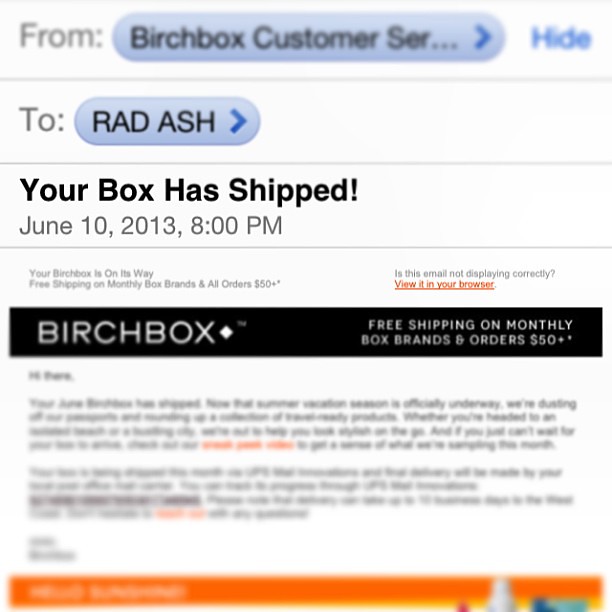The image is a screenshot of an email from Birchbox customer service to a recipient named Rad Ash. The main body of the email reads, "Your box has shipped. June 10th, 2013, at 8pm," indicating that the order has been dispatched. The email features a prominent Birchbox banner stating, "Free shipping on monthly box brands and orders of $50 and more." Most of the text in the email is blurred out, likely for privacy reasons. At the bottom of the email, there is a small section of text in tiny font that includes a message for visual issues with a line reading, "Is this email not displaying correctly? View in your browser," highlighted in red and underlined. Additionally, there's a black box towards the bottom with "Birchbox" written in white font alongside a diamond symbol following the "X." The entire email is standard in layout, with most of its content obscured, focusing on the shipping notification and promotional offers.